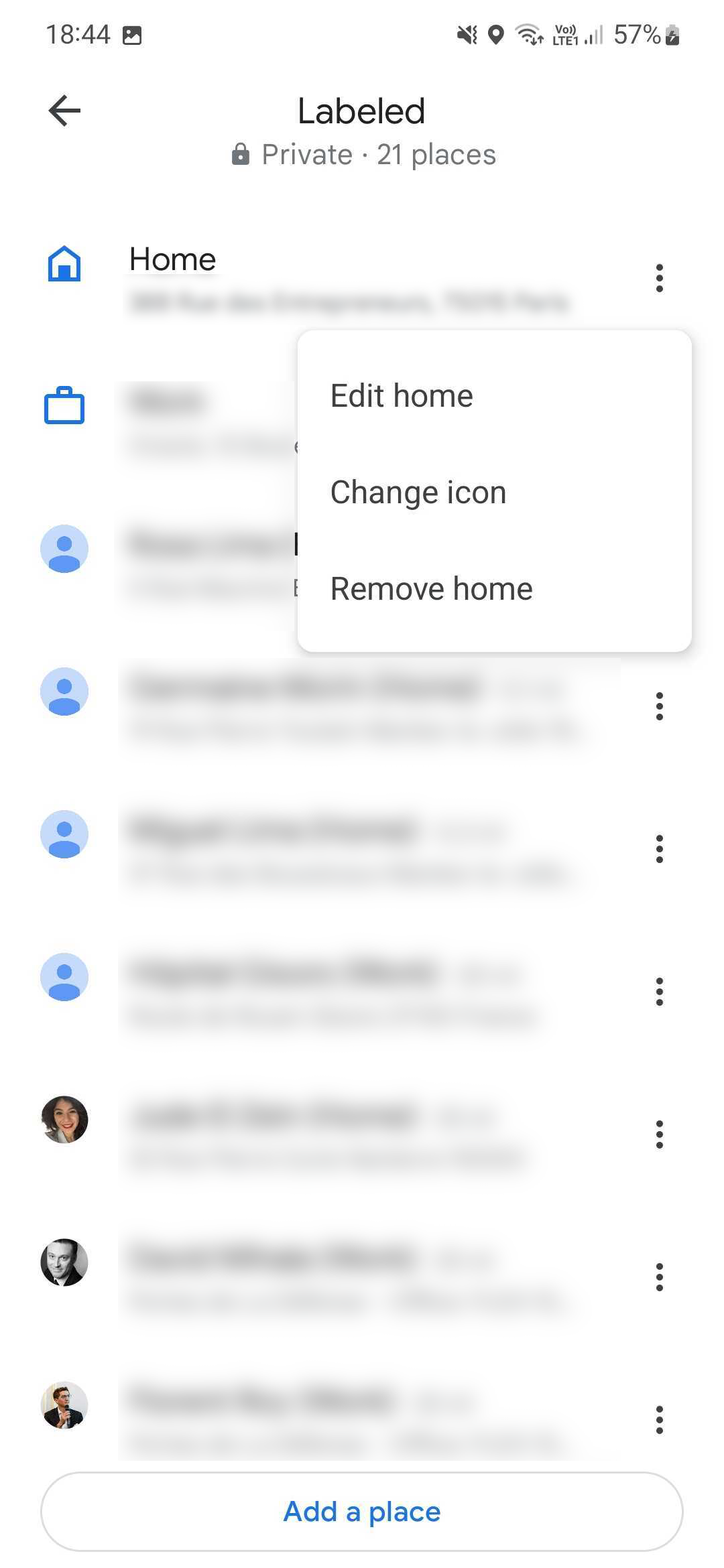The screenshot displays a smartphone screen at 18:44 hours with a location pin, two out of four signal bars, and a battery level of 57%. The top menu bar includes a black arrow pointing to the left. The main screen features a header with the label "Private 21 places." Below this header, a section labeled "Home" is represented by a home icon and a briefcase icon.

On the left side of the screen, there are four generic profile pictures followed by three real profile pictures, which are too small to identify. Each profile picture line on the far right side includes a vertical ellipsis (three dots). 

In the top-right corner, a pop-up box displays options to "Edit Home," "Change Icon," and "Remove Home." At the very bottom of the screen, there is an oblong-shaped box with blue text in the middle that reads "Add a place."